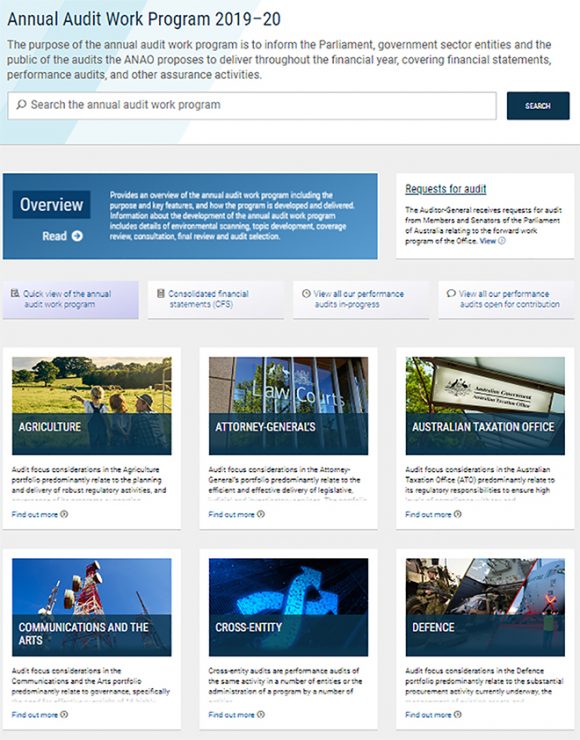The image captures a website dedicated to the Annual Audit Work Program for 2019-20. In the upper left-hand corner, the title "Annual Audit Work Program 2019-20" is prominently displayed. Beneath the title, there is a detailed blurb explaining the program's objective: "The purpose of the Annual Audit Work Program is to inform the Parliament, Government, Sector, and Entities, and the public of the audits the ANAO proposes to deliver throughout the financial year. These audits cover financial statements, performance audits, and other assurance activities." 

At the center of the page, there is a search bar labeled "Search for the Annual Audit Work Program," accompanied by a search button to its right. Directly below the search bar is a section titled "Overview," though the accompanying text is somewhat blurry. On the same line to the far right, there is an option labeled "Request for Audit," which also features a brief, blurry description underneath.

At the bottom of the page, there are two rows of thumbnail images, each row containing three thumbnails, making for a total of six thumbnails.